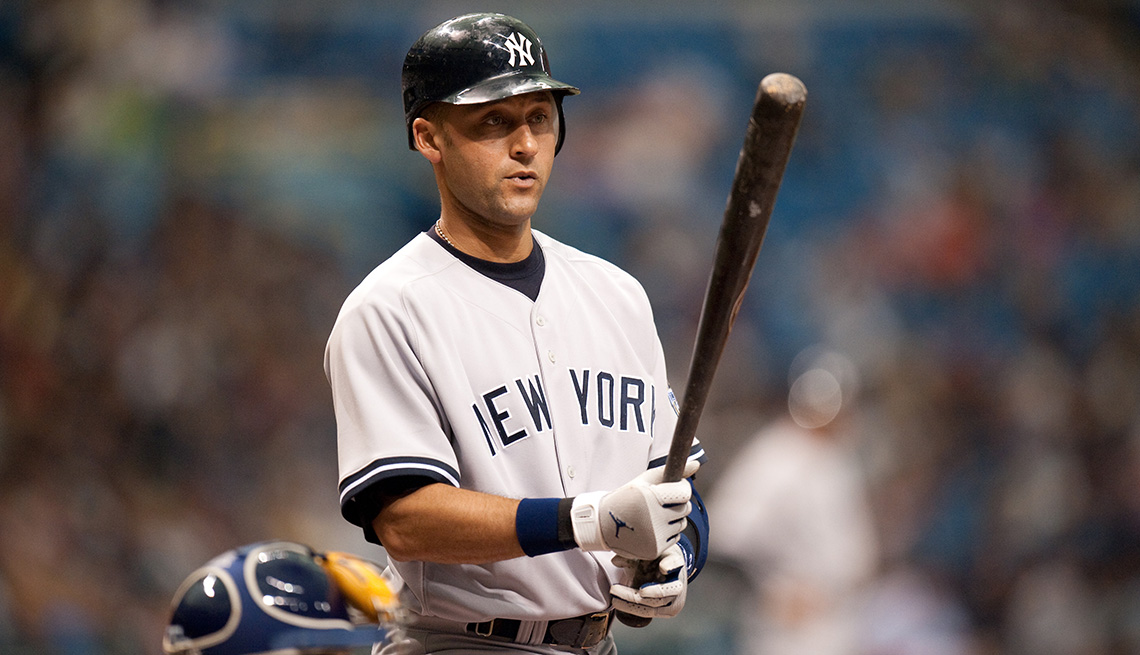In this detailed photo, we see a New York Yankees player, possibly Derek Jeter or Carl Ripken Jr., though there is some uncertainty. The player is outfitted in full baseball attire, including a prominent black safety helmet with the iconic New York Yankees emblem centered on the front. He is wearing a gray uniform shirt emblazoned with the word “New York” in blue letters across the chest, with blue trim around the sleeves, and underneath, a black or dark-colored t-shirt. He holds a well-worn bat in his gloved hands, preparing to step up to bat. The player's gloves are blue and white, and he faces to the right side of the image. Behind him, slightly out of focus, there's a catcher's helmet, indicating the presence of a catcher crouched down, though the details are unclear due to the blur. The background is filled with indistinct, blurry figures, suggesting a stadium with fans in the stands, adding to the anticipation and ambiance of the moment.